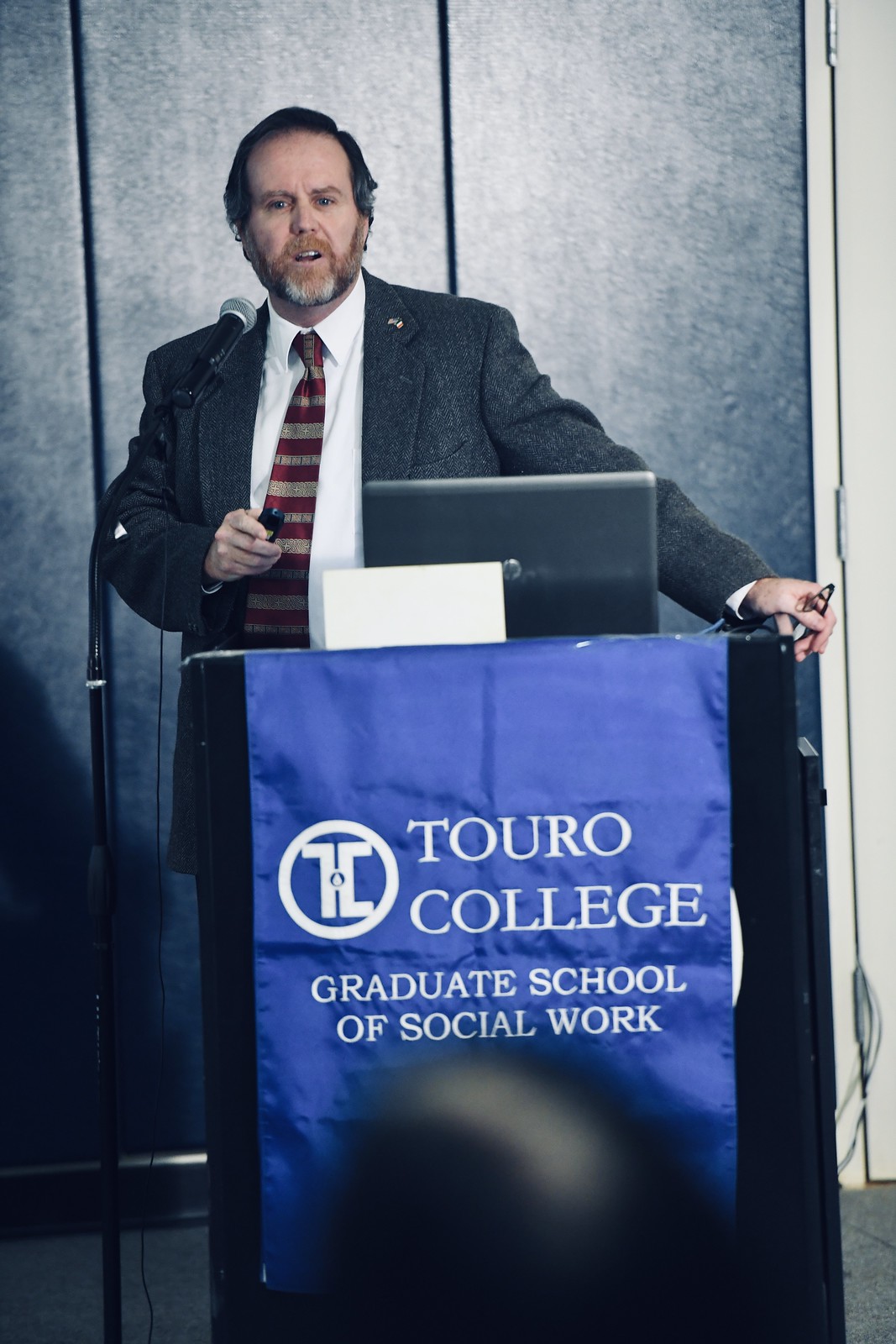The image shows a man standing behind a podium, facing slightly to the right. He is dressed in a gray tweed suit jacket, a white shirt, and a red and gold striped tie. He has short brown hair with hints of gray, accompanied by a small gray beard and a reddish mustache. His left hand, which is holding a pair of glasses, rests on the edge of the podium, while his right hand holds a small black device, possibly a laser pointer, in front of his torso. The podium features a prominent blue banner that reads "Touro College Graduate School of Social Work" with the college emblem on the left. An HP laptop is also placed on the podium. Behind the speaker, the backdrop is a wall composed of vertical gray panels. A microphone on a stand is positioned in front of him. In the foreground, slightly out of focus, the top of a spectator's head is visible, indicating an audience is present during his speech.